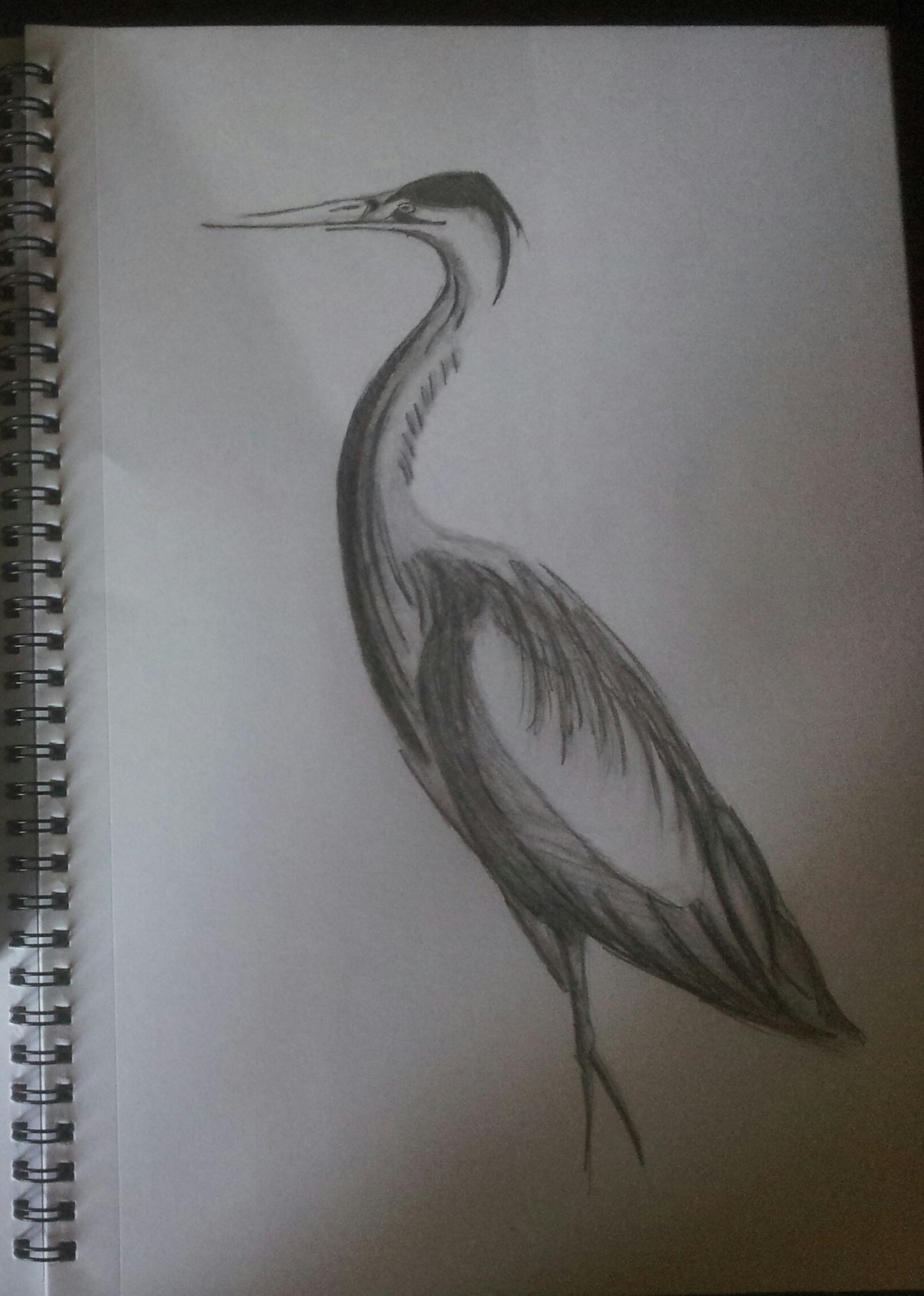A detailed charcoal pencil drawing on white paper captures the graceful figure of a crane. Standing upright, the bird gazes upwards and towards the left, creating a sense of poised alertness. The crane's left leg is positioned vertically, supporting its body, while the right leg angles subtly behind, adding a dynamic element to its stance. Tucked in close to its body, the wings showcase a fullness and rounded shape that gently taper near the tail. The slender neck curves with a gentle upward arc before reconnecting to the body, leading to a long, narrow, and pointed beak. The meticulous use of charcoal emphasizes the intricate textures of the feathers and the elegant structure of the crane.